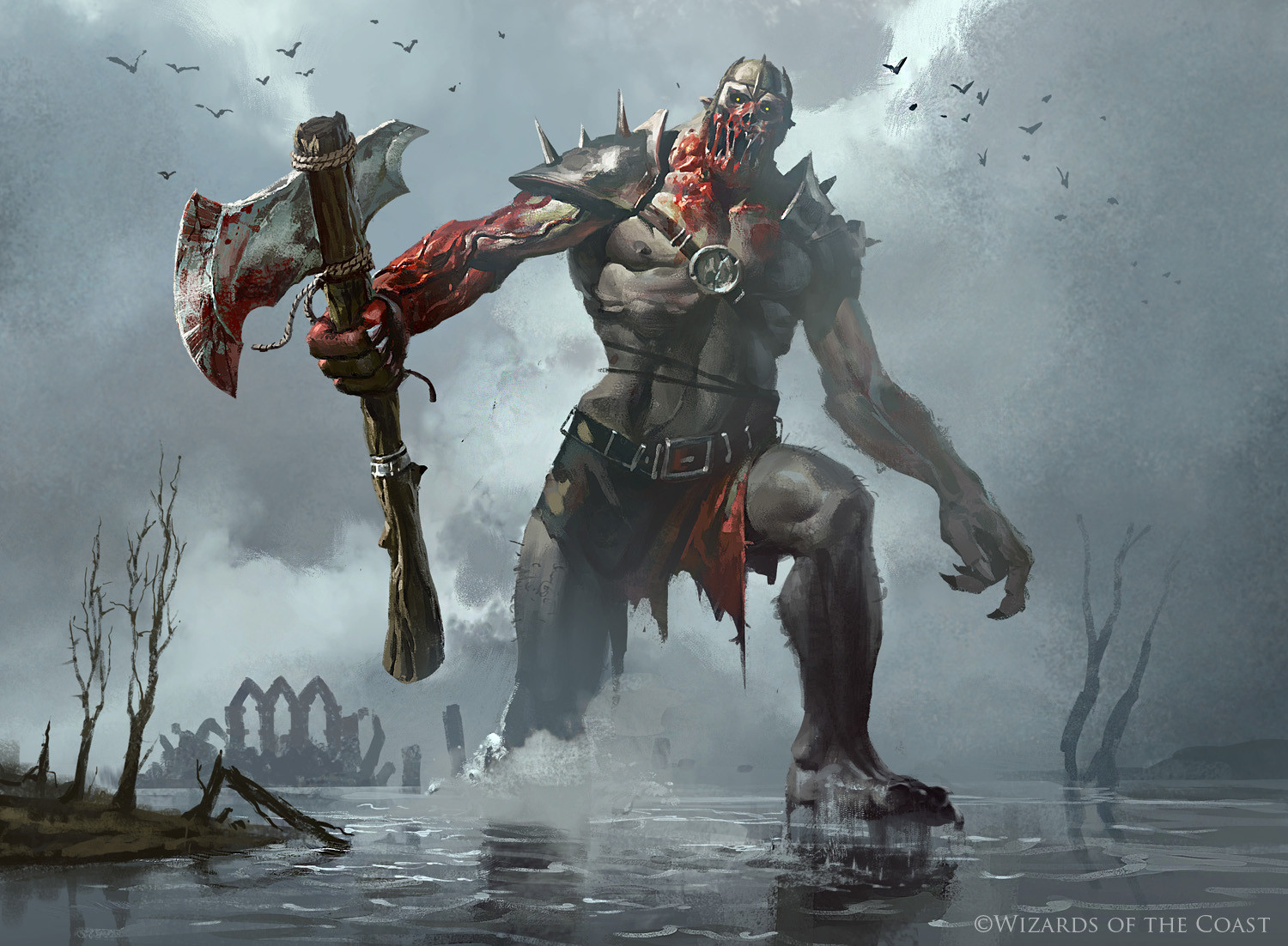This illustration, likely inspired by a fantasy book or film, showcases a dark and foreboding scene. The bottom corner bears the logo of Wizards of the Coast, hinting at its source. The atmosphere is thick with murky gray clouds, casting an eerie light over the landscape. A flock of black birds flies ominously high in the sky, enhancing the sense of impending doom. In the foreground, twisted, dead-looking trees emerge from dark waters, standing as sentinels over the desolation. 

The ruins of a stone building with crumbling arches loom in the background, adding to the scene's bleakness. From the water, a grotesque creature makes a dramatic entrance. Its appearance is terrifying, marked by spiky shoulder pads adorned with massive metallic spikes. A medallion rests on its chest, and a large belt with a square buckle hangs from its middle. Blood drips from its face, and its mouth is agape, suggesting it has just finished a brutal kill. The creature wields a massive axe, also stained with blood, indicating it is primed for further carnage.